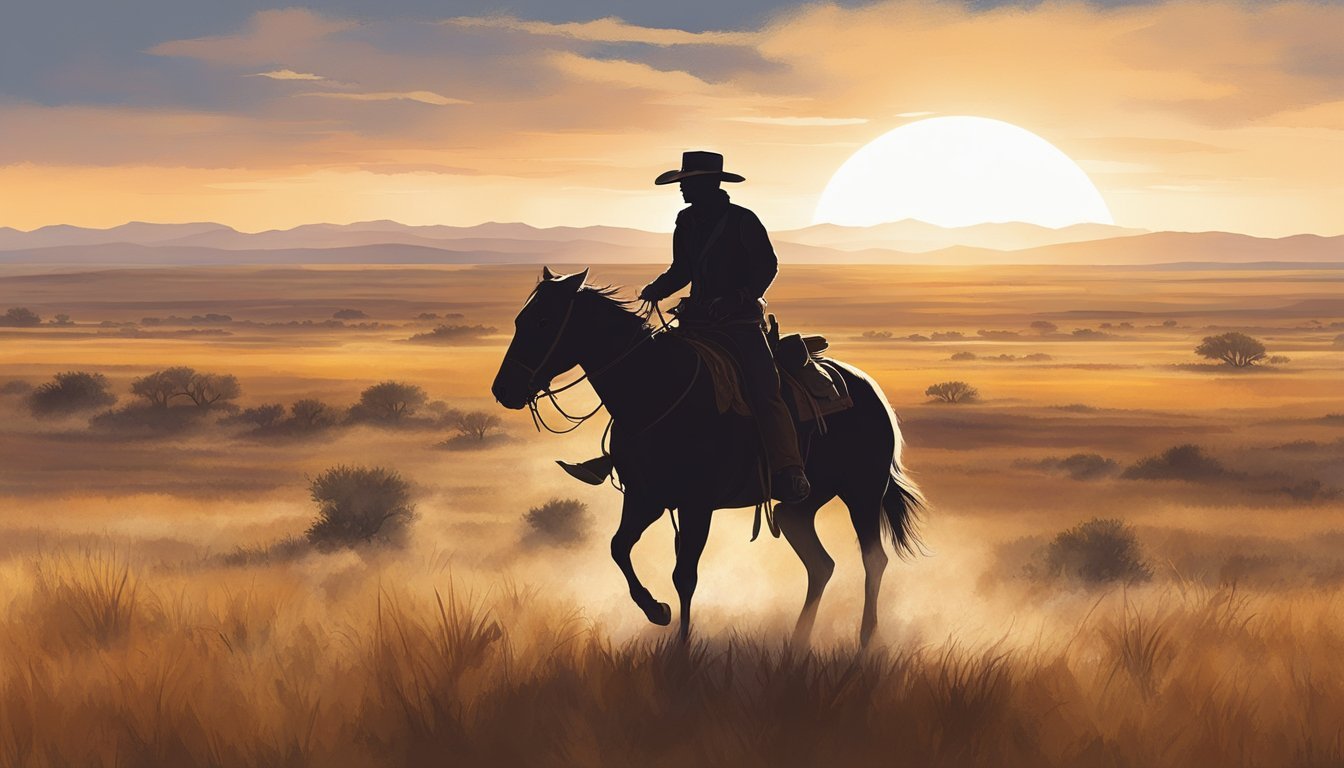The image is a captivating Western painting set in a dry, expansive plain bathed in golden hues. At the heart of this scene is a solitary cowboy riding a black horse, both depicted as shadowy silhouettes, making their attire and features indistinguishable. The cowboy is clad in traditional attire, complete with a black cowboy hat, and sits on a saddle as he rides across the dusty terrain, kicking up a trail of dust. 

In the foreground, the land is strewn with sparse green bushes and tall, golden-yellow grasses that wave gently. The vast landscape is painted with a gradient of colors, dark blue in the distance transitioning to various tones of orange and gold closer to the viewer. A line of mountains stretches from left to right in the background, creating a natural boundary for the plains.

The sky above is a stunning blend of white and blue clouds, softly illuminated by the top of the sun rising from the bottom right toward the top right. This rising sun casts an orange glow over the cloud cover and the rugged land below, painting a picture of both warmth and solitude in this quintessential Western scene.